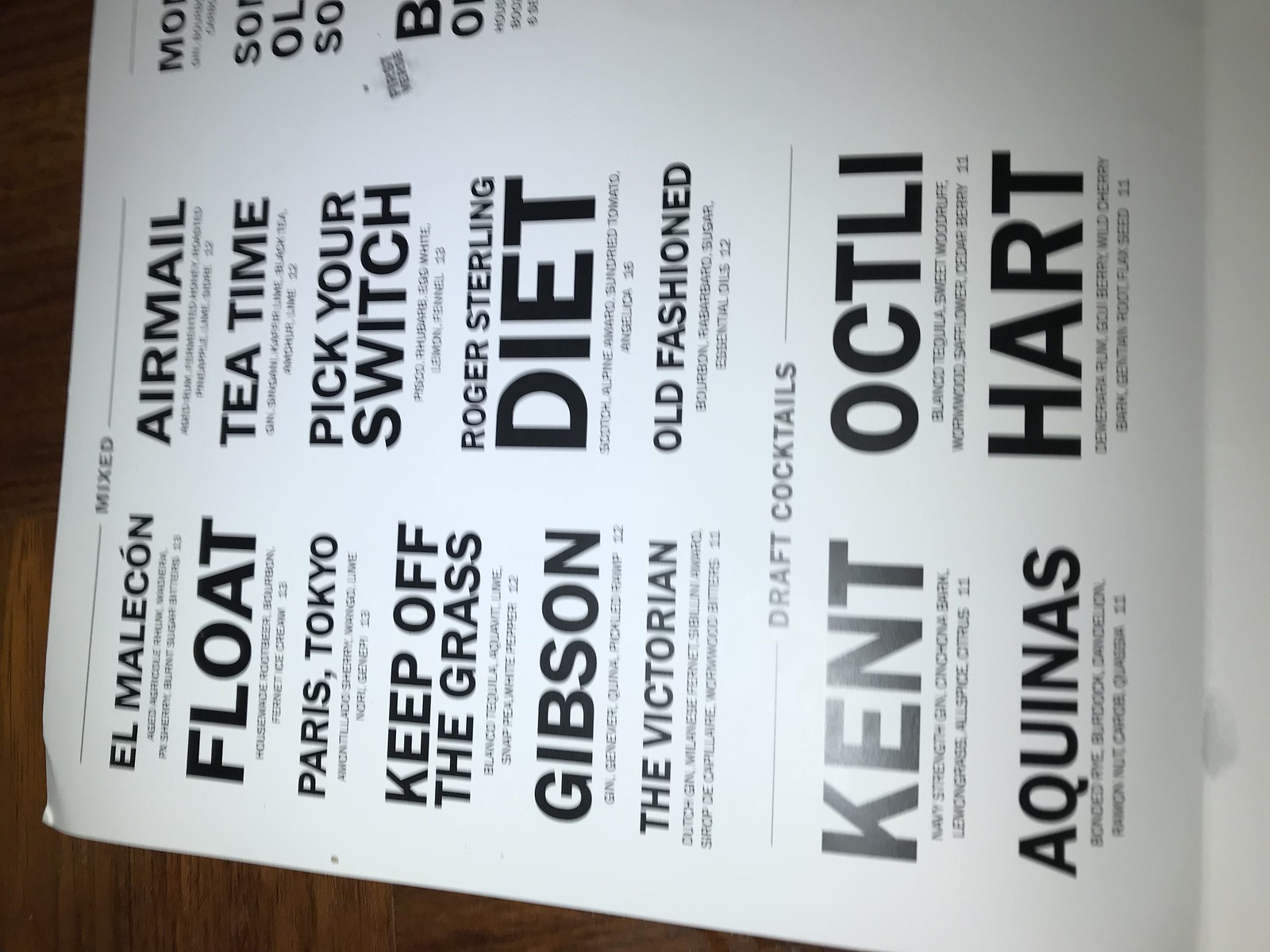The image shows a sideways-oriented menu, presumably for drinks, printed on a white piece of paper with black text. The menu is divided into two main sections: "Mixed" and "Draft Cocktails."

### Mixed:
1. **El Malecon**
   - (Details are illegible)
2. **Float**
3. **Paris, Tokyo**
4. **Keep Off the Grass**
5. **Gibson**
6. **The Victorian**

### Column under Mixed:
7. **Air Mail**
8. **Tea Time**
9. **Pick Your Switch**
10. **Roger Sterling Diet**
11. **Old Fashioned**
   - **Bourbon**, (Illegible), **Sugar**, **Essential Oils**
   - Price: **$12**

### Draft Cocktails:
#### Main Headings:
- **Kent**
- **Aquinas**
- **Octili (O-C-T-L-I)**
- **Hart (H-A-R-T)**

#### Example Under Octili:
- **Blanco Tequila**, **Sweet Woodruff**, (Illegible), **Safflower**, **Cedarberry**
- Price: **$11**